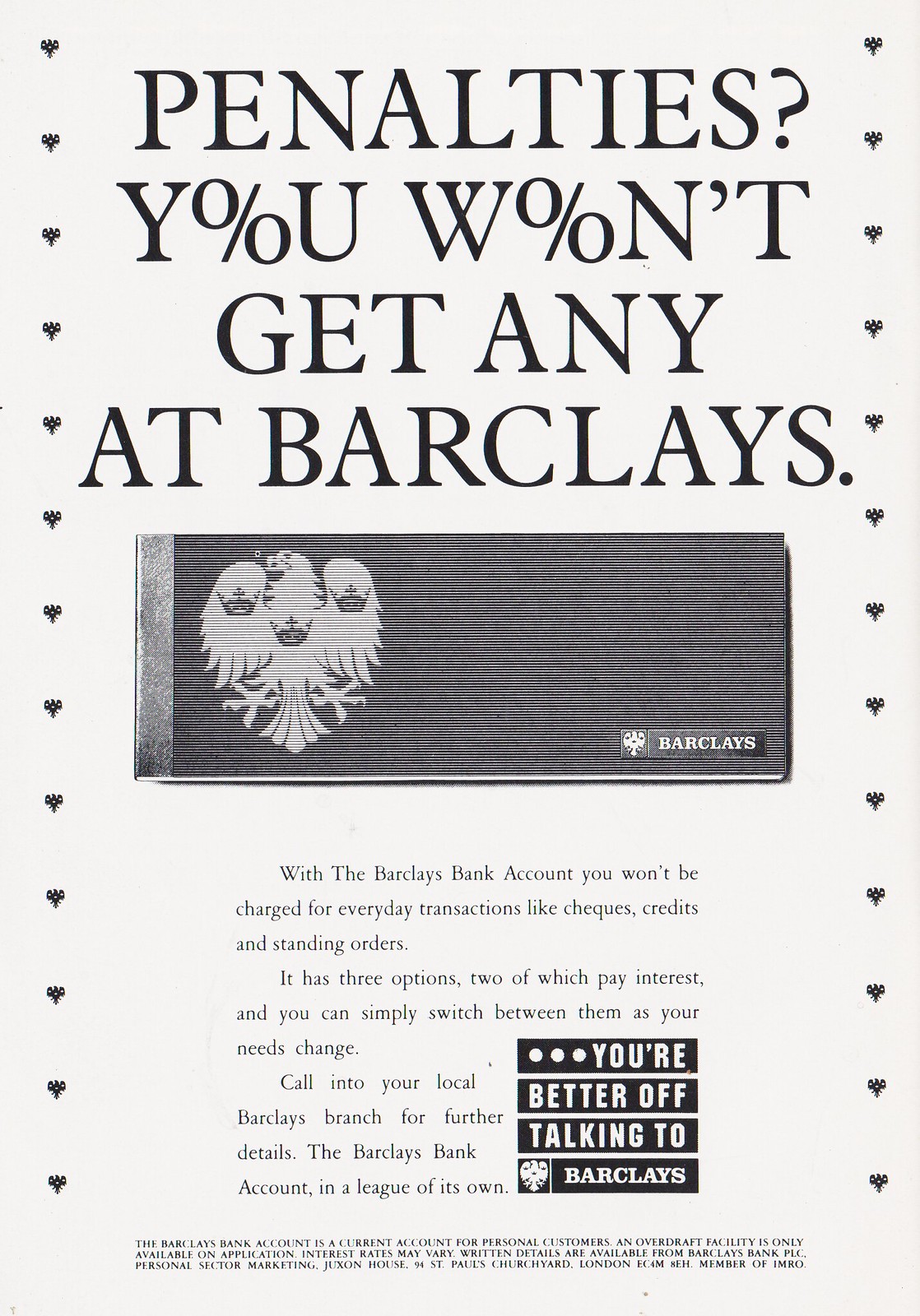The advertisement is a full-page ad for Barclays Bank, featured on an all-white background and likely found in a magazine or an official game day program. At the top, in large black font, it asks "Penalties? Y%U won't get any at Barclays," with the O's in the words "you" and "won't" replaced by percentage signs. Below this headline lies a regal logo of a three-headed eagle with two talons and a tail, accompanied by the word "Barclays." 

Further down, the ad features explanatory text detailing that with a Barclays Bank account, customers won't incur charges for everyday transactions such as checks, credits, and standing orders. The account offers three options, two of which accrue interest, allowing flexibility to switch between them as needed. Potential customers are encouraged to visit their local Barclays branch for more information. The text concludes with the slogan, "The Barclays Bank account, in a league of its own." Additionally, there's bold, black text stating, "You're better off talking to Barclays." The sophisticated layout is augmented by some indistinct vertical shapes along the sides, adding a subtle design element to the otherwise minimalistic page.